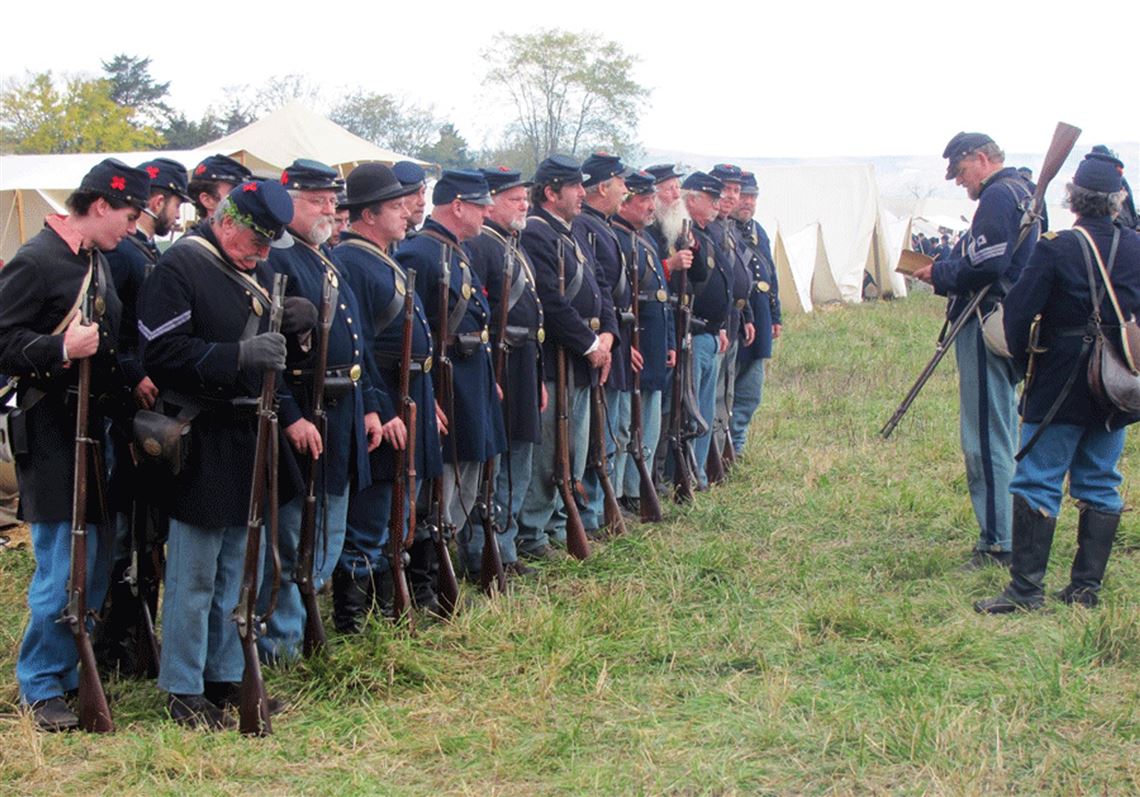In this detailed image, we see a well-organized group of Civil War reenactors dressed as Union soldiers. They are identified by their dark blue jackets with silver buttons, light blue pants, and matching blue caps. The soldiers are lined up in a grassy area, where white canvas tents and hints of trees in the background set the scene. Each soldier holds a single-action rifle or musket, standing loosely but uniformly focused in one direction. At the forefront, a leader or general, also in Union attire, is reading from a book with his rifle resting on his shoulder. This setting suggests an early morning, perhaps due to the faint fog visible in the air, implying preparations for a day of historical reenactment are underway.